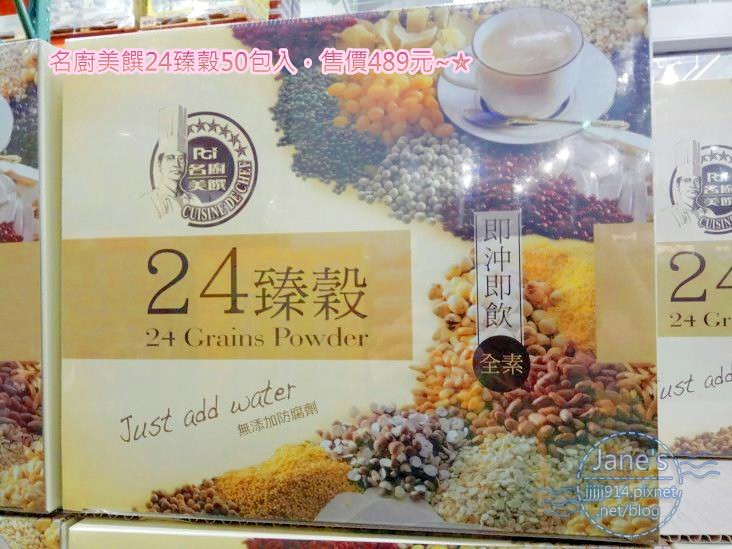This image captures a prominent box on a shelf, possibly in a supermarket in China, showcasing various types of grains. The box, which may be behind a reflective glass window or wrapped in shiny plastic, is notable for its detailed packaging and vibrant visuals. At the top left corner, there is a logo featuring a Chinese chef wearing a chef's hat, enclosed in a circle, with six stars and the phrase "Cuisine de Chef" at the bottom. The central part of the box displays "24 grains powder" in a gold rectangle with black font, followed by instructions to "just add water". Encircling a white teacup with a black rim and a silver spoon resting on a matching saucer, the front of the box illustrates various grains, hinting at the product's natural and diverse ingredients. Chinese characters dominate the packaging, along with numbers such as 24, 50, and 489 visible on the top left, making it somewhat challenging to determine the complete product description and ingredients.